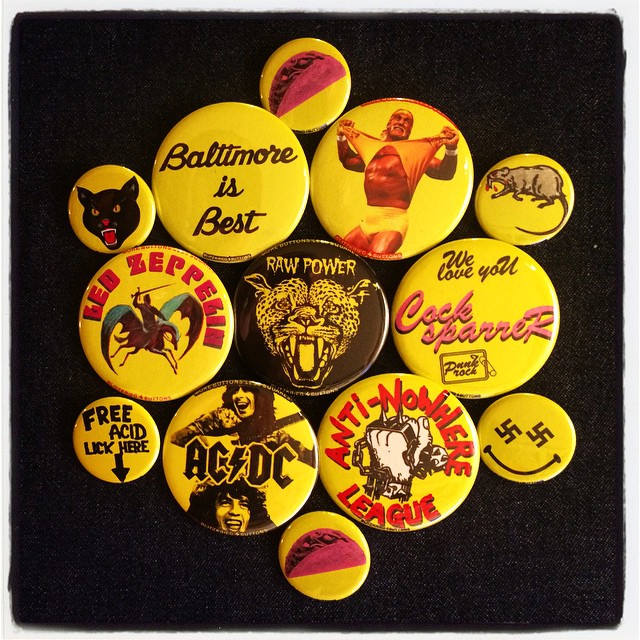This is a detailed photograph of a button collection displayed on a piece of black square cloth, likely a jacket or fabric. The collection comprises thirteen pins of varying sizes, predominantly featuring a light yellow base color with black elements, though there are some exceptions. Positioned in a visually striking manner, these pins encapsulate an eclectic blend of 80s pop culture. 

At the top, a small pin showcases a red taco, while the adjacent small pin displays a black leopard or panther. Below, a larger pin proudly declares "Baltimore is best" in bold text. Nearby, another pin immortalizes wrestler Hulk Hogan ripping his shirt. 

Among the collection, there is also a small pin featuring a rat and another large one emblazoned with the phrase "Raw Power" alongside the image of a leopard. Moving leftward, one pin depicts a man riding a winged horse, possibly referencing Led Zeppelin imagery. 

One small pin provocatively directs "Free Acid lick here" with an arrow pointing downward, while another large pin shows the iconic ACDC logo alongside band members. Further down, an Anti-Nowhere League pin displays a red font and a fist graphic. 

Subtly positioned small pins include one with a smiley face using swastikas for eyes, highlighting the diverse and often controversial nature of 80s pin culture. The collection is anchored by a single central pin with a black background featuring yellow text and graphics. This assortment of pins, varying from images of animals like rats and leopards to bold textual statements and representations of musicians and wrestlers, creates a vivid homage to the vibrant and dynamic spirit of the 80s.